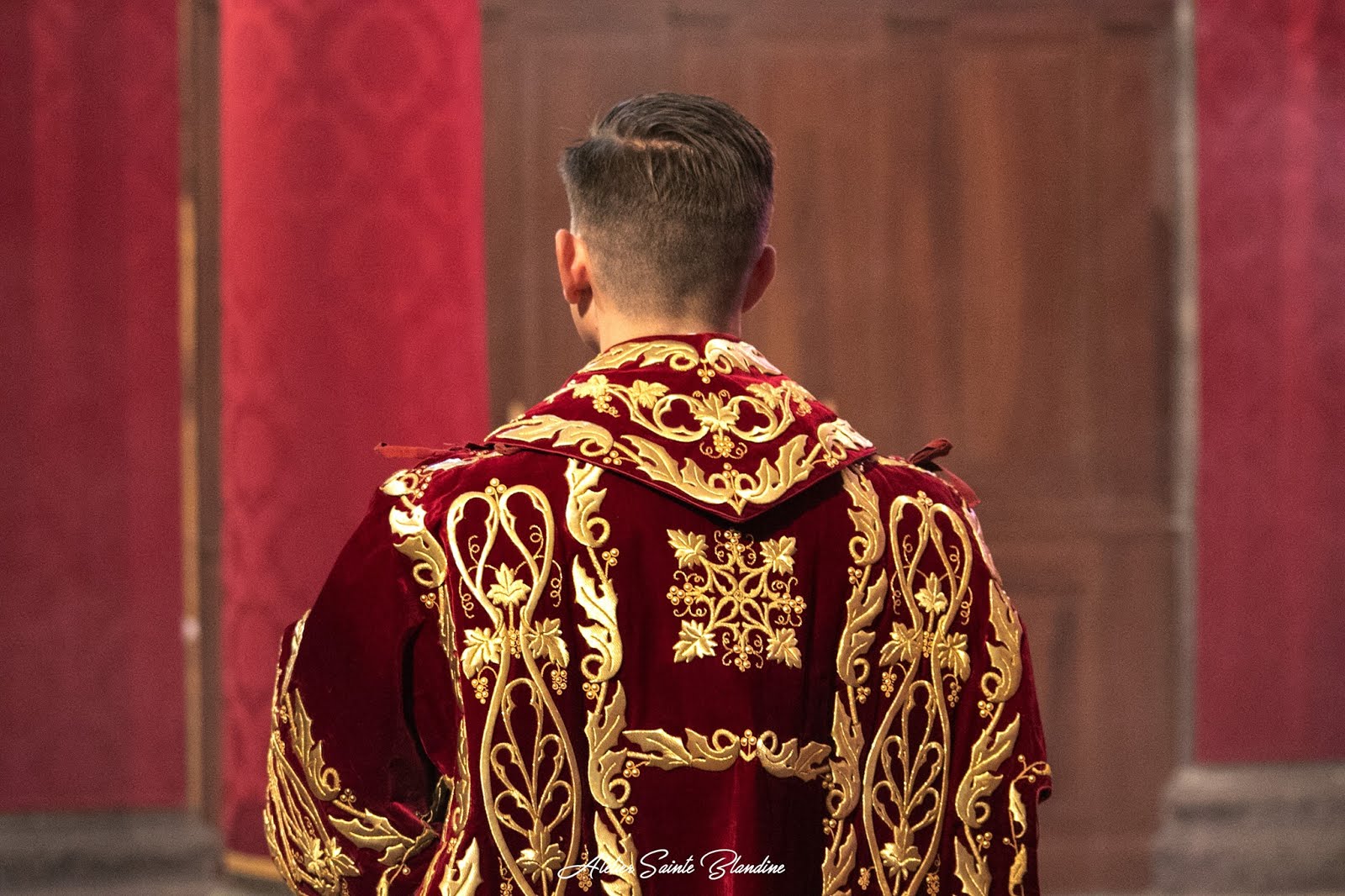The image depicts the back of a man, likely a religious figure officiating a church service, based on his ornate and ceremonial attire. He is dressed in a luxurious red velvet robe adorned with intricate gold embroidery. The robe features various detailed design elements, including leaves, shapes, and trims. Notably, there are two prominent golden bars running down from his shoulders, connected by additional gold embroidery, forming a square pattern in the center of his back. The man's close-cropped, dirty blonde hair is parted on the left, and his ears are visible. He stands before a backdrop comprising red panels or draperies and what appears to be a large wooden door. The lower part of the image contains partially obscured cursive text, potentially saying "Saint Valentine's" or "sainty, blandine," though some letters are difficult to discern. Overall, the detailed vestments and setting suggest a religious or ceremonial context within a church.